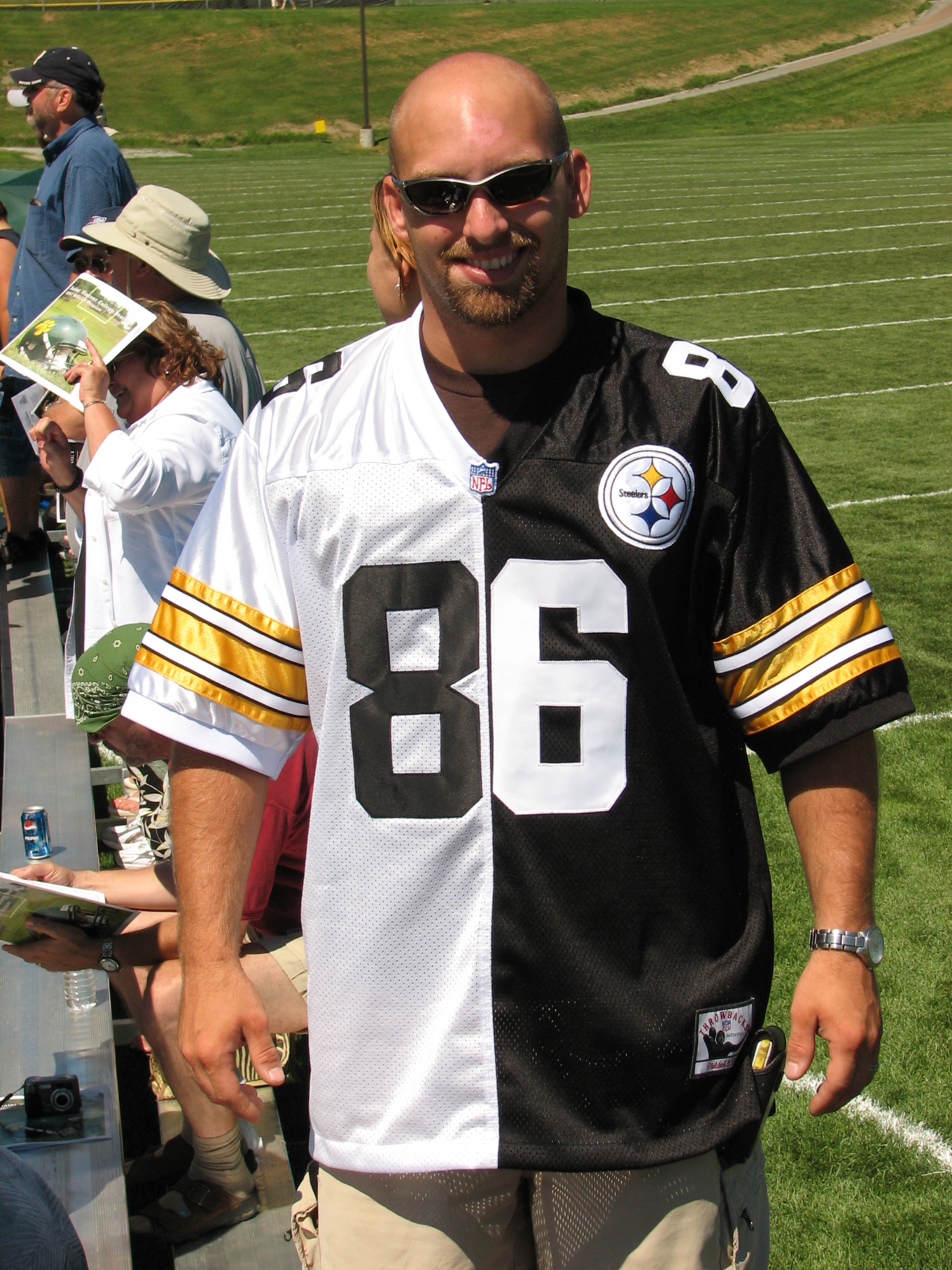In the image, we see a bald man wearing dark sunglasses and smiling at the camera while standing on a football field. He sports a distinctive Pittsburgh Steelers jersey featuring the number 86, with the left half of the shirt in white and the right half in black; the digits are inversely colored. The NFL logo is prominently displayed in the middle of the collar, while each sleeve is adorned with gold and white bands. His small beard and mustache, light brown in color, accompany his goatee, adding to his friendly appearance. The man is also wearing a silver watch on his left wrist and khaki beige shorts. The background reveals a grass-lined field, likely belonging to a high school, middle school, or elementary school, rather than an official Steelers' arena. To his left, several spectators, possibly parents, are gathered in the bleachers, suggesting they are either watching or preparing for a game.